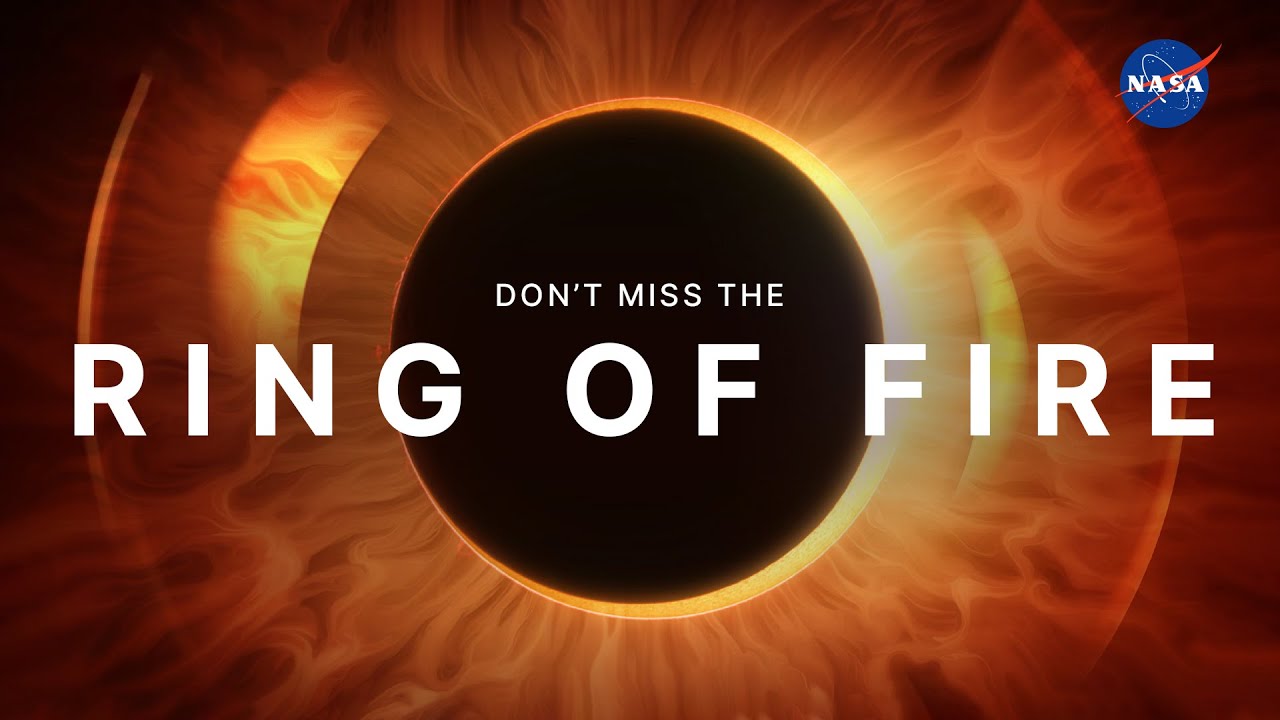The photograph is a contemporary NASA advertisement, structured horizontally and incorporating a vivid, digitally-rendered eclipse as its central focus. The top right corner features the NASA logo, anchoring the viewer's attention. In the center of the image is a black circle representing the moon, surrounded by a bright yellow ring, simulating the "ring of fire" effect seen during certain solar eclipses. Radiating outward from this central point are vibrant shades of orange and yellow, suggesting flames or solar rays. The text in the advertisement is split into two parts: "don't miss the" in small letters across the eclipse photograph, followed by the large, bold phrase "ring of fire," spanning the image. This design, likely intended for a digital platform like a website banner, aims to remind viewers not to miss an upcoming eclipse event.